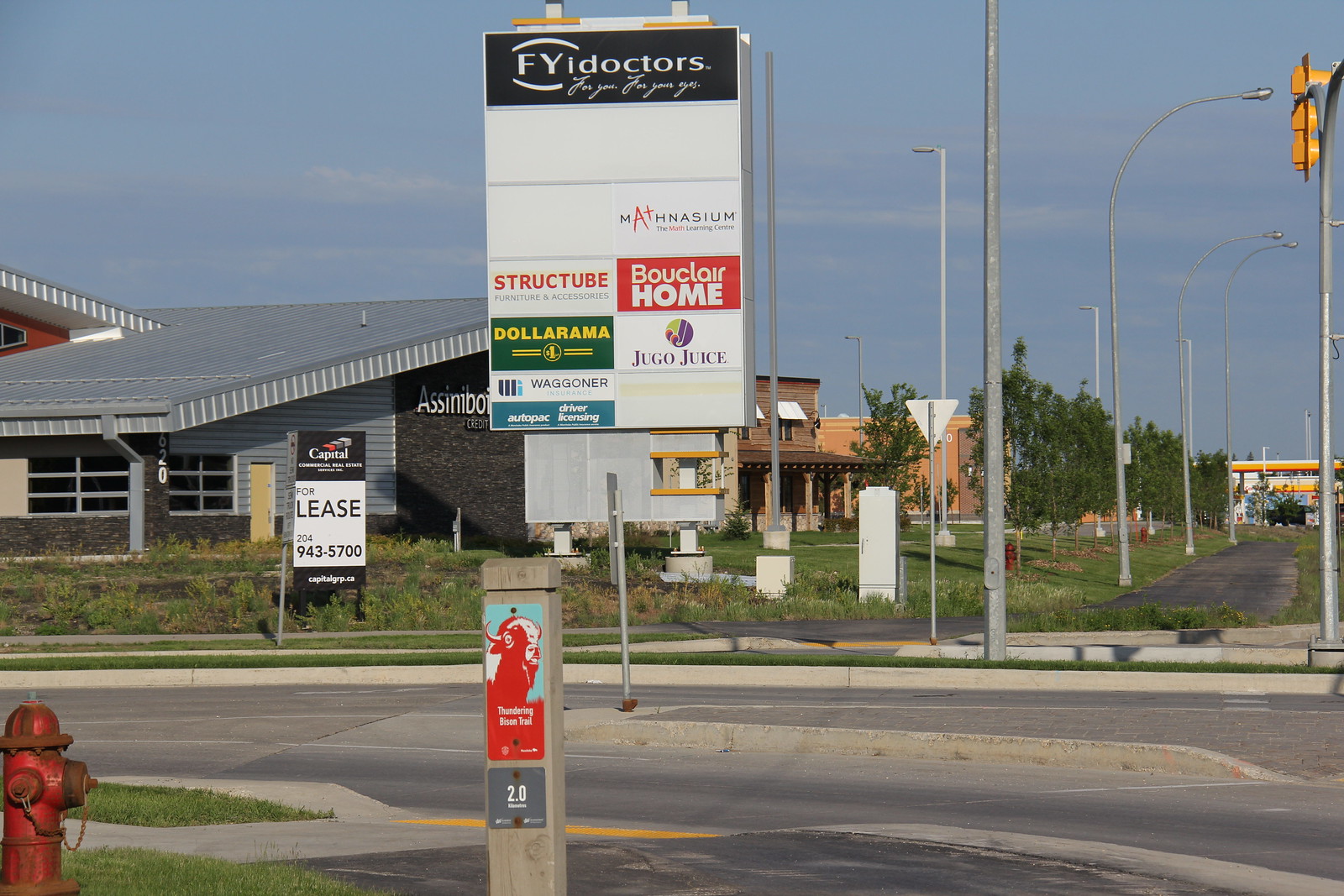This photograph captures a street mall from a corner viewpoint, displaying a detailed urban scene. In the foreground, on the lower-left corner, there's a prominent red fire hydrant. A crosswalk leads to a triangular median in a divided road. Across the street, an imposing sign lists various stores: at the top is "FYI Doctors," followed by a blank slot, then "Manhasium," "Structure," "Buclair Homes," "Dollarama," and "Jugo Juice."

Behind the sign, a large shop with a gray triangular roof and dark gray outer walls dominates the scene, leading to more brown-colored shops within the mall area. Scattered along the street are multiple lamp posts, adding character to the suburban shopping locale. Additional smaller buildings and a lease sign with white borders and black lettering can be seen further back, enhancing the depth of the scene. The blacktop sidewalk extends into the distance, guiding the viewer's eye toward further structures and activity in this bustling area.